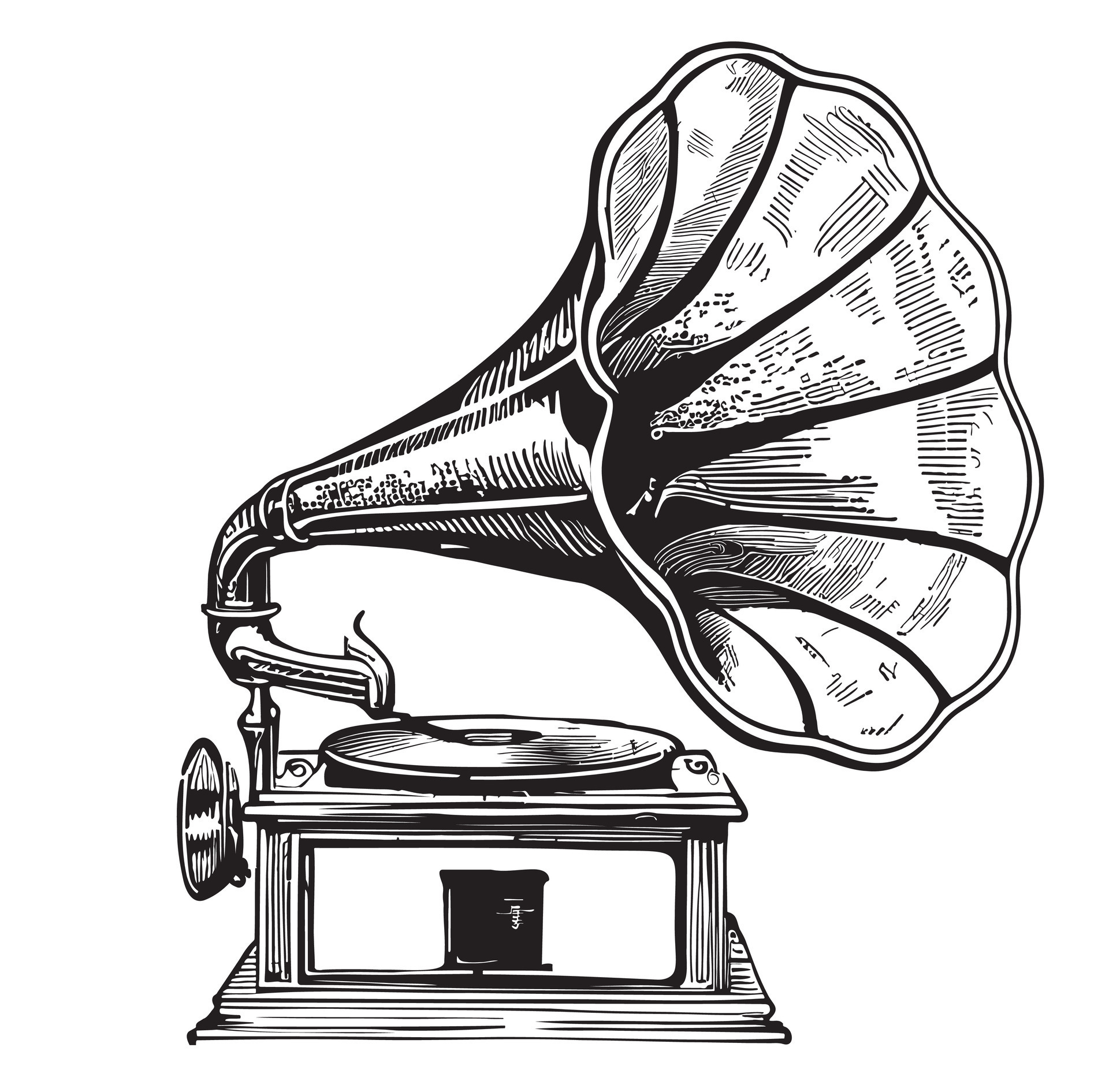The image is a detailed black and white etching of a vintage phonograph, commonly known as a gramophone. The background is stark white, highlighting the intricate design of the phonograph. Central to the image is a large, flower-shaped horn that extends down to the needle, which rests on a circular disc platter holding a vinyl record. This setup is mounted on a square platform containing the phonograph's mechanics and controls, with visible knobs and a switch. The whole apparatus is perched on a substantial wooden base. The etching employs variable-spaced lines to indicate different color intensity values, adding depth and texture to the monochromatic sketch. The horn, dominating the composition with its size and ornate detailing, is the focal point of the image.